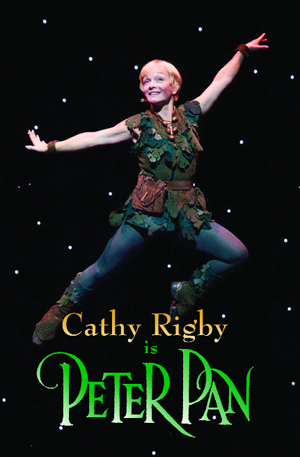The image is an advertisement for a Broadway production featuring Kathy Rigby as Peter Pan. Kathy Rigby is depicted flying through the air with her arms stretched out, in a vibrant and dynamic pose with one leg out and one knee up. She wears a sleeveless vest embellished with green leaves, a brown belt with a small red pouch, and dark blue or black tights. Her mid-calf boots are greenish-brown with leaf decorations above them. She also has leather wristbands and a very short, bob-style blonde haircut, with a joyous smile on her face. The background is black, dotted with white stars that enhance the magical atmosphere of the scene. The text at the bottom of the image features her name, "Kathy Rigby," in a yellowish-white gradient, and below it, the words "is Peter Pan" appear in a green-to-white gradient font.